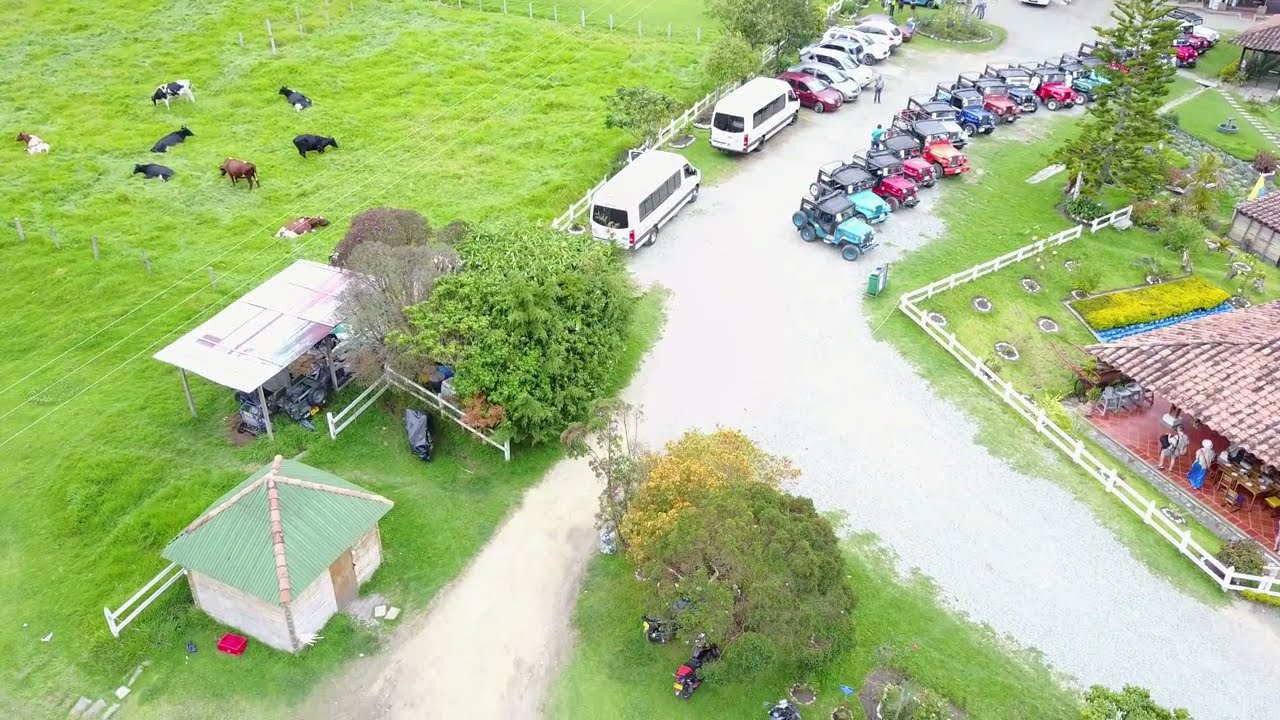This aerial daytime photograph captures a lively gathering at a scenic cattle ranch. The focal point is a large home with a distinctive red tile roof, encircled by a white wooden fence. Parked in front of the house, on a gray gravel driveway lined with trees, are numerous vintage Jeeps, specifically old-style CJ5s and CJ7s from the 1970s and 1980s, alongside a mix of modern sedans. To the right of this scene, catering vans are strategically positioned, indicating the event is well-catered.

Adjacent to the house is a sprawling grassy field where assorted cattle, including different colored cows—black, brown, black and white, and brown and white—are either grazing or resting. On this side, a small hut with a green roof is also visible, adding to the rustic charm. There’s a covered pavilion under which various equipment is parked.

Further to the right of the parking area, several golf carts in vibrant colors—turquoise, red, and blue—are neatly arranged. Another pavilion, likely for event attendees, features tables, chairs, and people milling about underneath. This pavilion, made of red brick with a red shingle top, is also encompassed by a white fence, tying back to the main house’s aesthetic. The photograph, taken from a high vantage point, reveals a detailed and bustling celebration, set against the backdrop of the picturesque and functional elements of a working ranch.